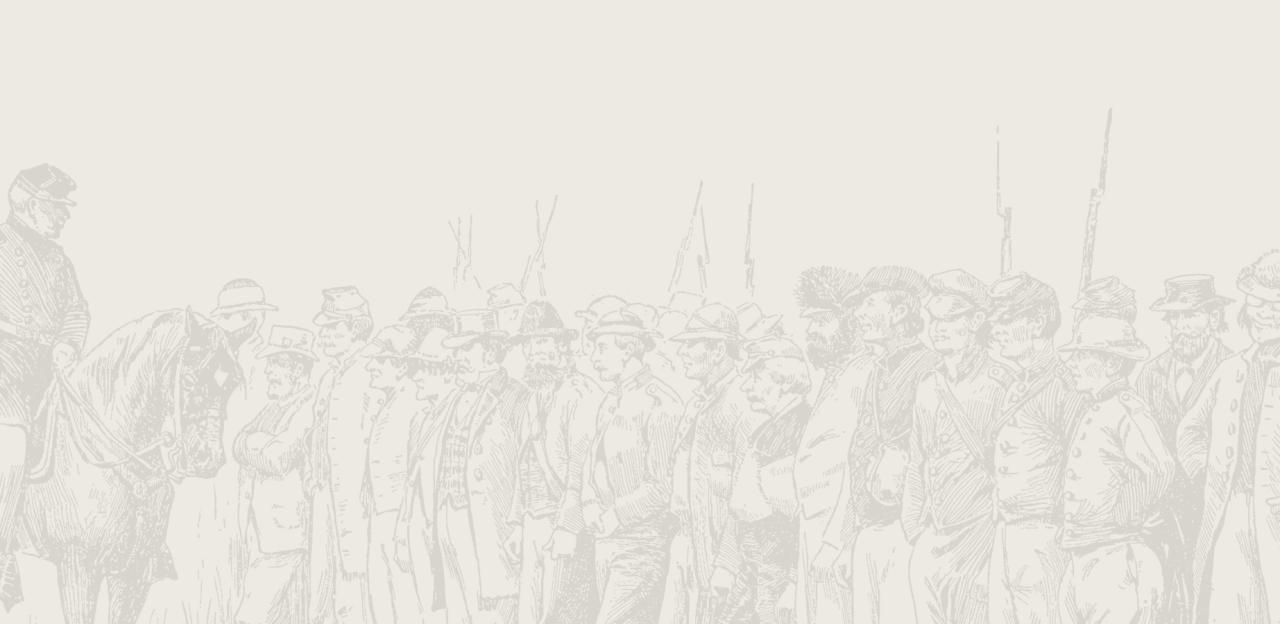The image, resembling a faint tracing covered by opaque tracing paper, depicts an illustrated scene of Civil War soldiers. On the left side is a cavalry officer mounted on a horse, possibly representing Southern troops due to their ragtag appearance. The group consists of various men, differing in age, some quite old. A few soldiers wield weapons with bayonets, while many appear unarmed. There are around two dozen men, each wearing different head coverings, most hats, and none with helmets. Their attire varies; some don short coats and uniform bottoms, others don long coats or civilian clothes. The overall impression is of a diverse and haphazardly equipped Confederate unit.